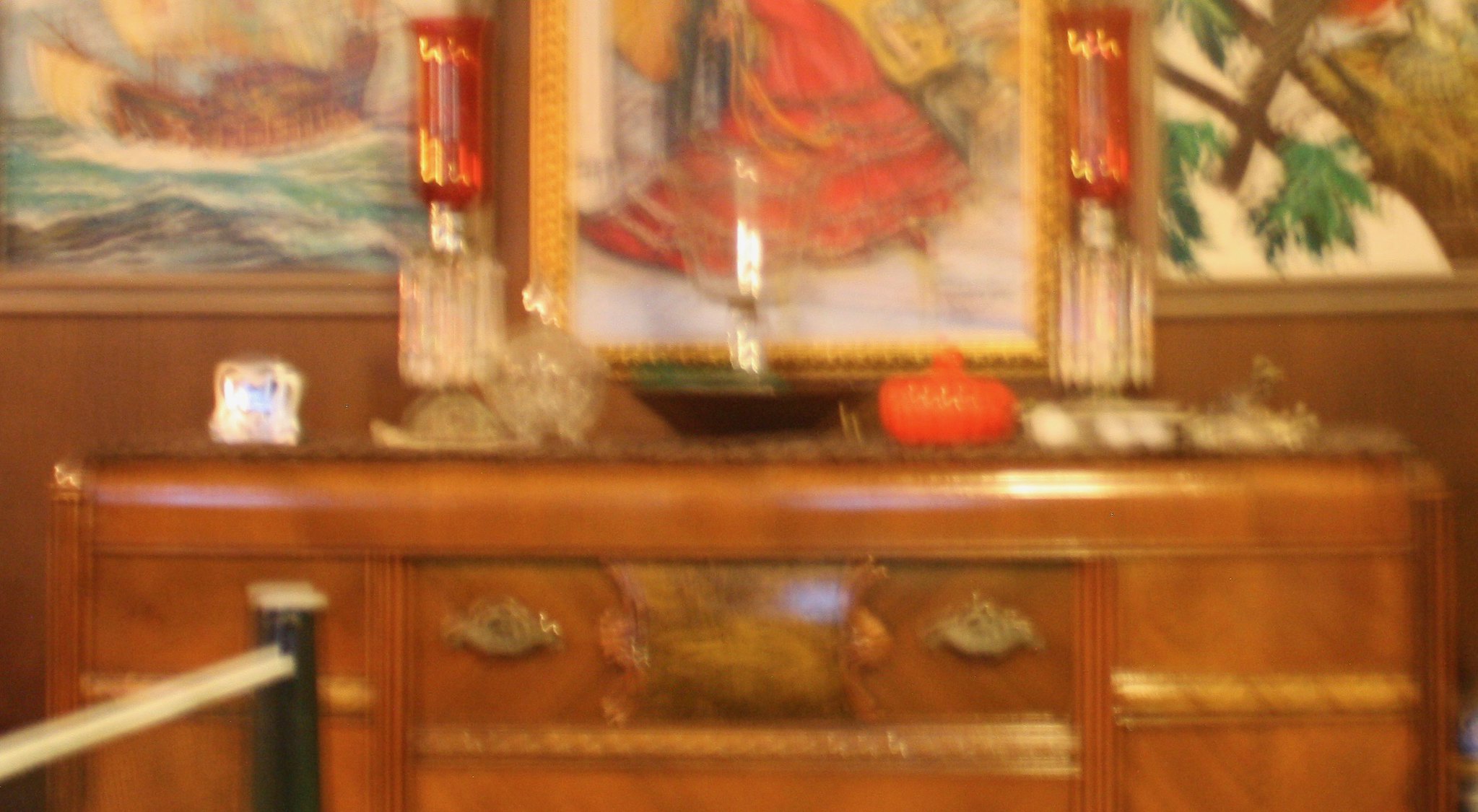This blurry image depicts a large, wooden dresser with a distinctly brown hue, composed of three sections with two on the sides and a central, largest drawer. The drawers are separated by wider horizontal pieces of wood. The central drawer is notable for its ornate design, featuring two large metal handles and a decorative square made of wood. On top of the dresser sits an array of glass items, including two glass vials placed symmetrically on the left and right. These vials have clear glass bottoms and red, tulip-like shapes at the top, resembling small lamps. Additionally, in the middle of the dresser, there is a black bowl holding lit candles. The wall behind the dresser showcases three artworks with elegant borders: the left painting appears to depict an antique wooden ship on a blue ocean, the center one seems to portray a girl in a red dress, and the right one looks like a bird perched in a tree. The backdrop is a plain, dark brown wall, darker than the dresser itself. The photo suggests a museum setting, indicated by a black pole with a line, likely serving as a barrier to keep people at a distance.